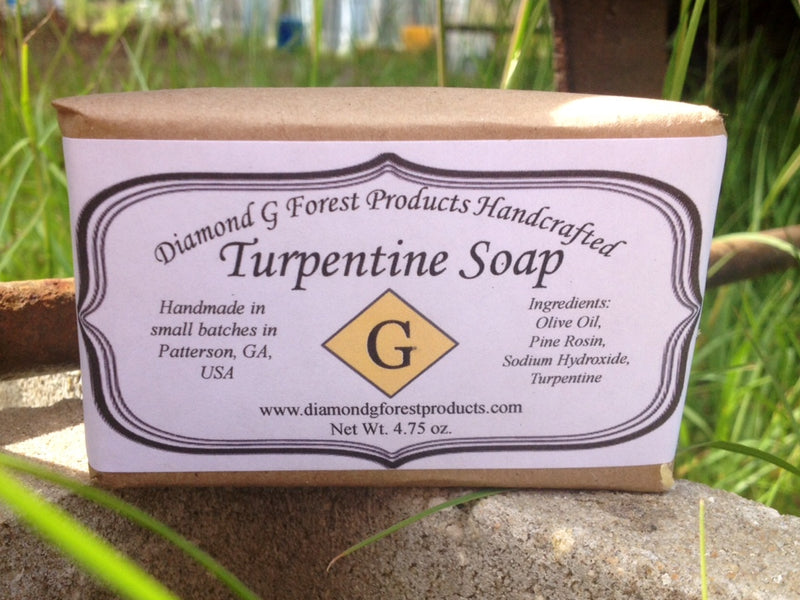This is a detailed close-up photograph of a bar of handcrafted turpentine soap. The soap is wrapped in brown cardboard paper and has a white label that stretches across the front. On the label, at the top, it says "Diamond G Forest Products Handcrafted" in an arched black font. In the middle of the label, prominently displayed in large black letters, it says "Turpentine Soap." Beneath this, aligned to the left, it reads "Handmade in small batches in Patterson, Georgia, USA," and to the right, it lists the ingredients: olive oil, pine rosin, sodium hydroxide, and turpentine.

Centered on the label is a yellow diamond-shaped emblem with a black capital letter "G." At the bottom of the label, it provides the website "www.diamondgforestproducts.com" and states the net weight of the soap as 4.75 ounces. The soap is positioned on a stone, outdoors, with a backdrop of grass, leafy plants, and a tree visible, suggesting a natural, sunny setting.